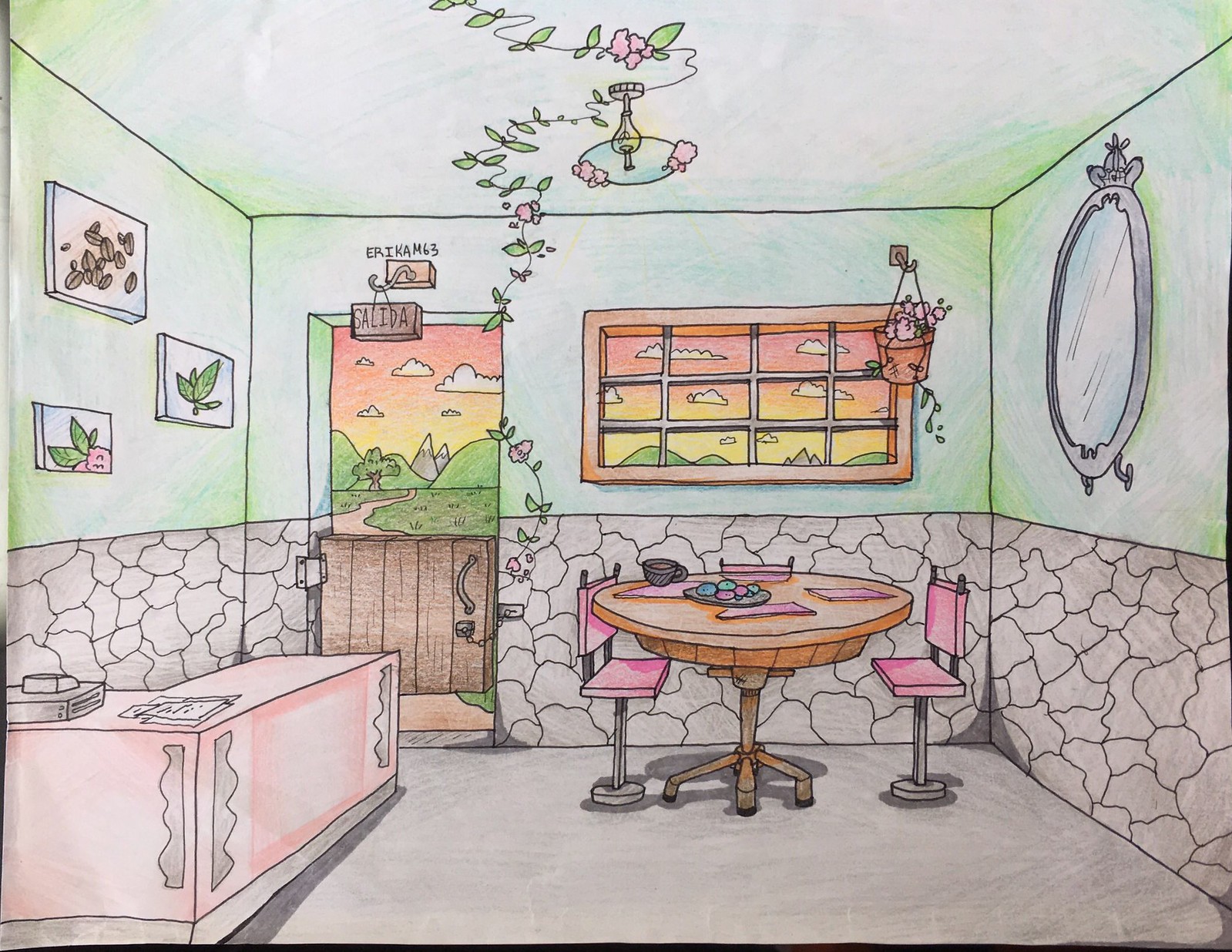This image is a color sketch of the inviting interior of a small, cozy restaurant or café. The artist has meticulously used colored pencils or watercolors to bring out the vibrant ambiance of the room. The right side features flagstone walls that go halfway up, transitioning to light green plaster towards the ceiling. A hanging lamp with a vine drapes centrally across the room, adding a charming touch.

To the left, there's a counter possibly holding menus, painted in a pink hue. Above it, the wall is adorned with various plant images and framed pictures, adding warmth and character.

Dominating the right corner of the room is a round table with a brown surface, set with four placemats and a single cup. The table is paired with two pink high-top chairs that resemble bar stools with seat backs, comfortably nestled under the table when not in use. There's also a large oval mirror enhancing the room's depth, reflecting the serene yet lively décor.

A half door and a swinging door with hinges and a handle lead to an alluring pathway. Beyond these doors, a picturesque walkway opens up to green hills and majestic snow-capped mountains under a radiant amber-reddish sky dotted with puffy white clouds, suggesting a sunset.

Above the door is inscribed “Salida” and “Erica M63,” further personalizing this quaint and colorful space. The overall effect is a very pleasant, detailed depiction of a charming and inviting room that blends the comfort of home with the vibrancy of a favorite local café.